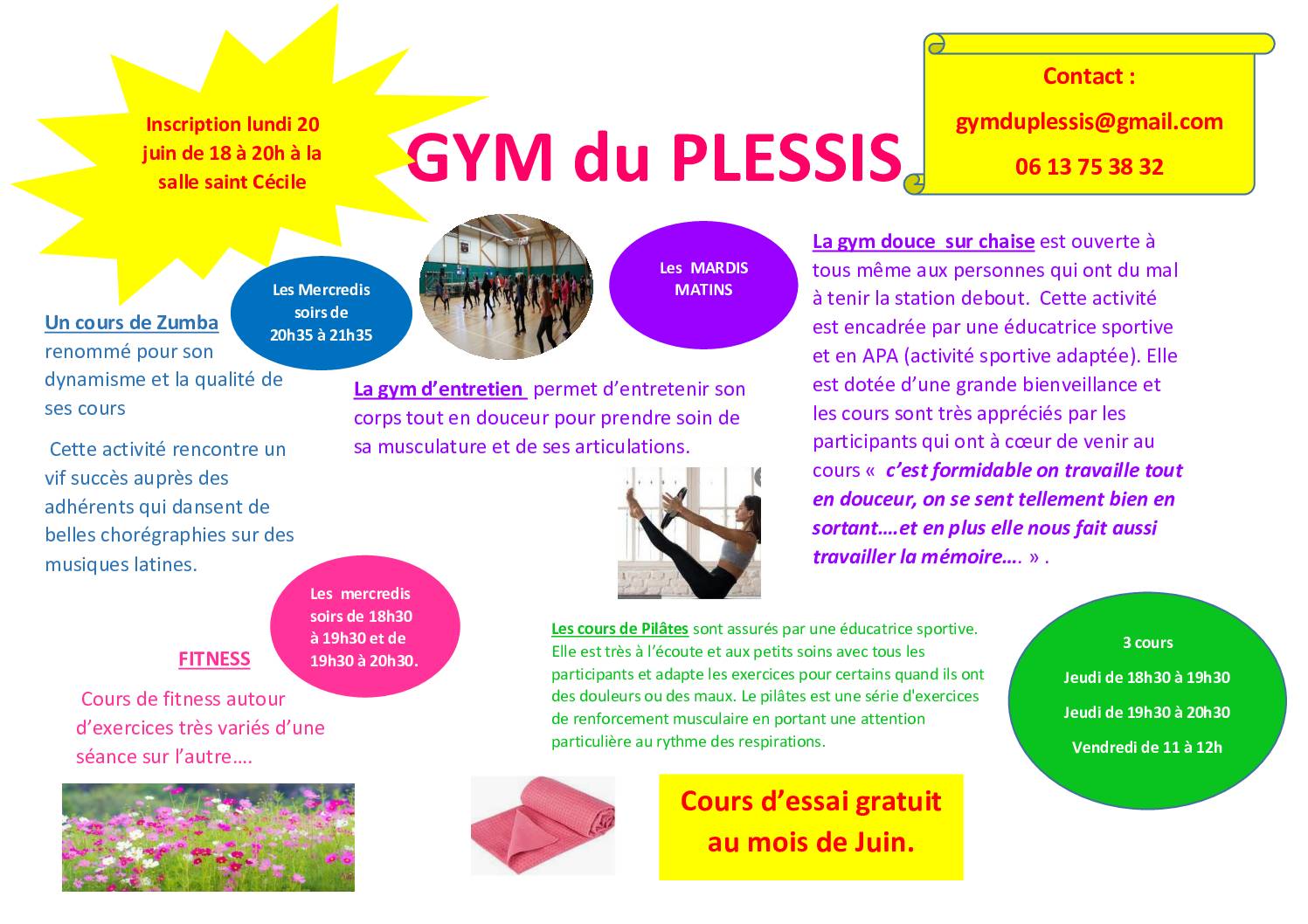The advertisement is for "Gym du Plessis," a gymnasium, and is entirely written in French. In the upper left, a sunburst icon highlights event dates. The top right features contact information: an email address (gymduplessis@gmail.com) and a phone number (0613753832). The flyer details the gym's offerings, including Zumba, Pilates, a basic gym area, and fitness classes, with days and times provided for each activity in various colored circles scattered across the page. A central image shows a woman in tights and a form-fitting long-sleeved top performing aerobics with a weight. Below, in the center, another woman is depicted doing Pilates. A blue circle provides details about these classes. At the bottom, a promotional offer for June is indicated, accompanied by an image of wildflowers and a mat. Each section is color-coded, with green, pink, purple, and yellow text and shapes organizing the information visually.